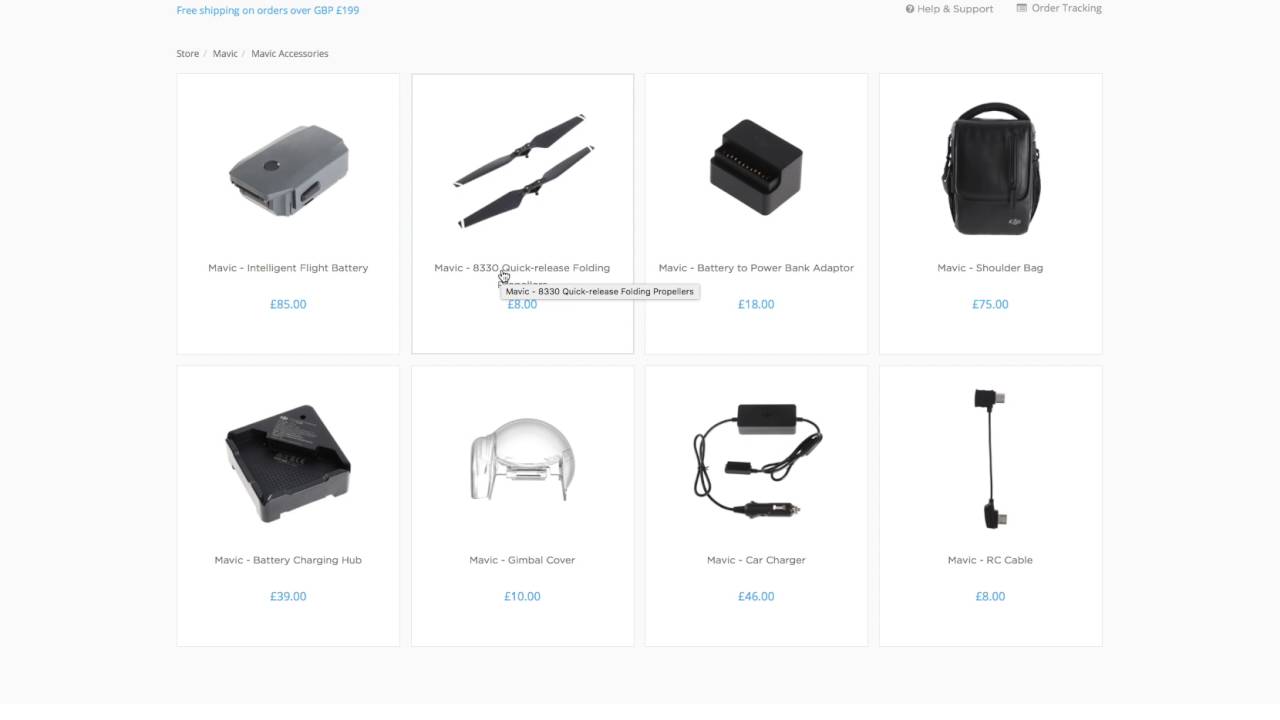This detailed image showcases an assortment of Mavich products along with their prices. In the top left corner, there's a banner highlighting "Free Shipping on Orders of £199." Featured in the image are: 

- Mavich Intelligent Flight Battery priced at £85. 
- Mavich 8330 Quick Release Folding Propellers available for £8. 
- Mavich Battery to Power Bank Adapter for £18. 
- Mavich Shoulder Bag costing £75. 
- Mavich Battery Charging Hub priced at £9. 
- A Gimbal Cover for £10. 
- A Car Charger available at £6.

The background text includes "Store" and "Mavich Accessories," indicating these items are part of the Mavich brand accessory lineup.